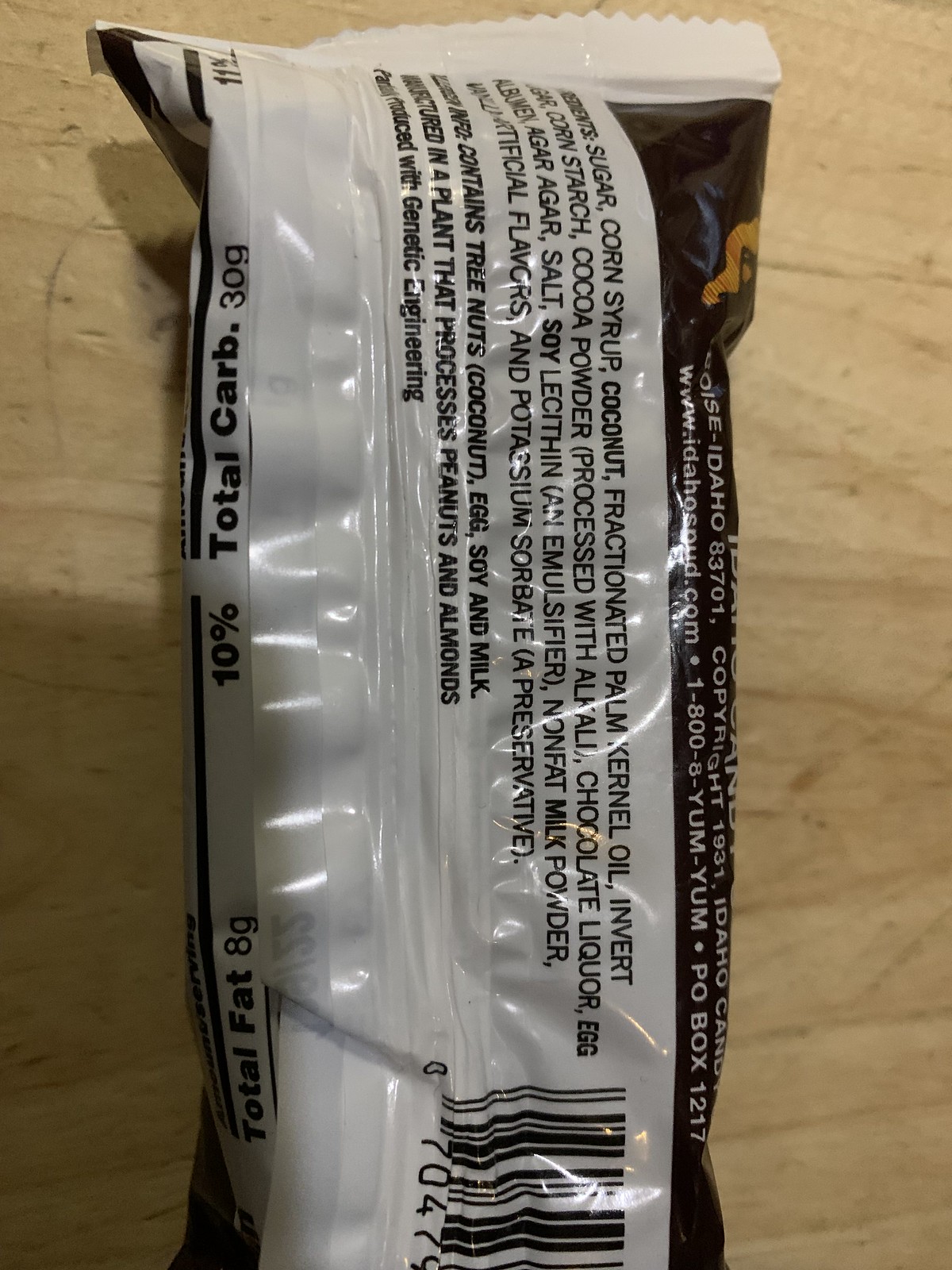The image captures the back of a small packet from Idaho Candy, likely containing a confection known as Idaho Spud. The packet, set against a light cream-colored wood grain table, features a detailed ingredients list: sugar, corn syrup, coconut, fractionated palm kernel oil, invert sugar, cornstarch, cocoa powder (processed with alkali), chocolate liquor, egg albumin, agar agar, salt, soy lecithin, nonfat milk powder, artificial flavors, and potassium sorbate. The nutrition facts indicate that the product contains 8 grams of total fat and 30 grams of total carbohydrates per serving. A barcode is also visible at the bottom of the label, alongside a partial view of the nutrition information and a copyright date of 1931. The prominent label "Idaho Spud" initially suggests a potato product, but the ingredients confirm it is a candy bar.